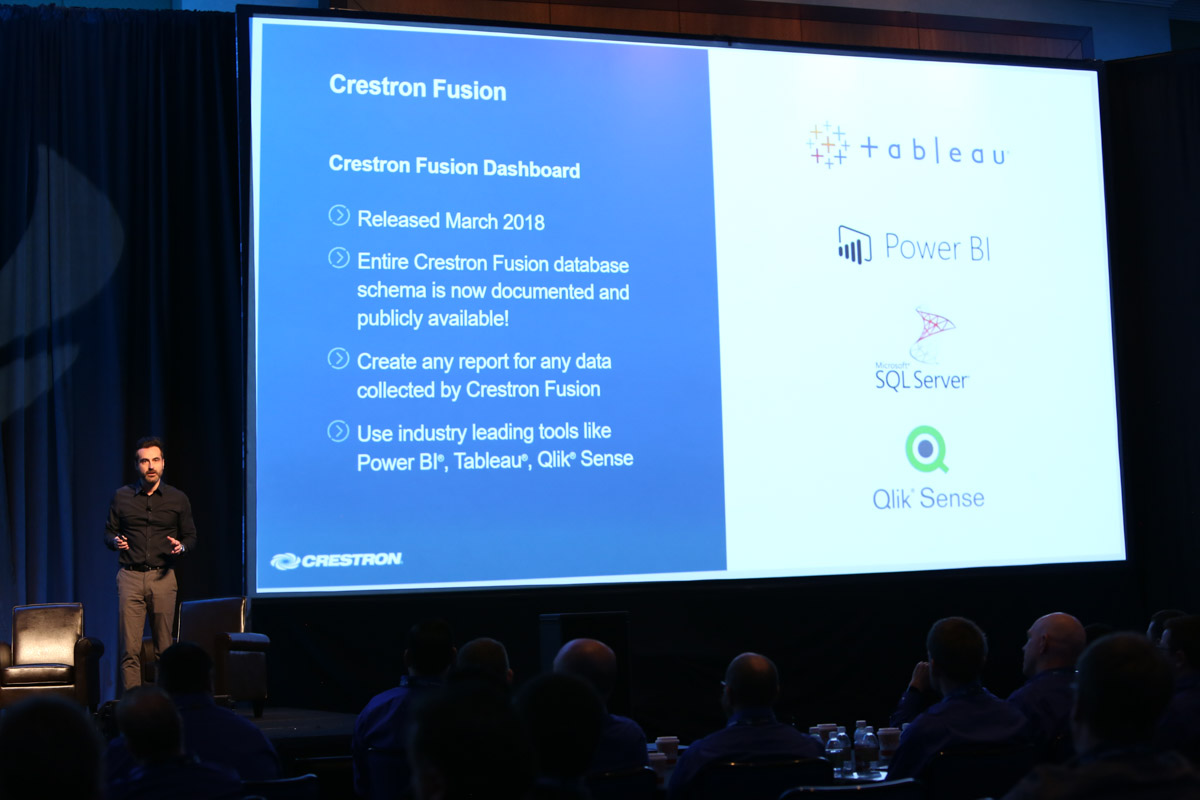The image portrays a man giving a presentation in the bottom-left corner of the frame. He has short dark hair, a beard, and is dressed in a black collared shirt and grayish tan pants. The setting includes a blue curtain behind him. He appears to be gesturing with his hands while addressing an audience dressed in business attire who are seated at tables adorned with water bottles. The audience is mostly in the dark while focusing on the speaker.

A massive screen dominates the right side of the image. The screen is split into two sections: the left half is blue with white text, and the right half is white with several logos. The text on the blue section reads, from the top: "Crestron Fusion," "Crestron Fusion Dashboard," "Released March 2018," "Entire Crestron Fusion database schema is now documented and publicly available," "Create any report for any data collected by Crestron Fusion," and "Use industry-leading tools like Power BI, Tableau, or QLIKSense." Adjacent on the white section, logos for Tableau, Power BI, SQL Server, and QLIKSense are lined up vertically. The photograph vividly captures the formal setting and the technological theme of the presentation.